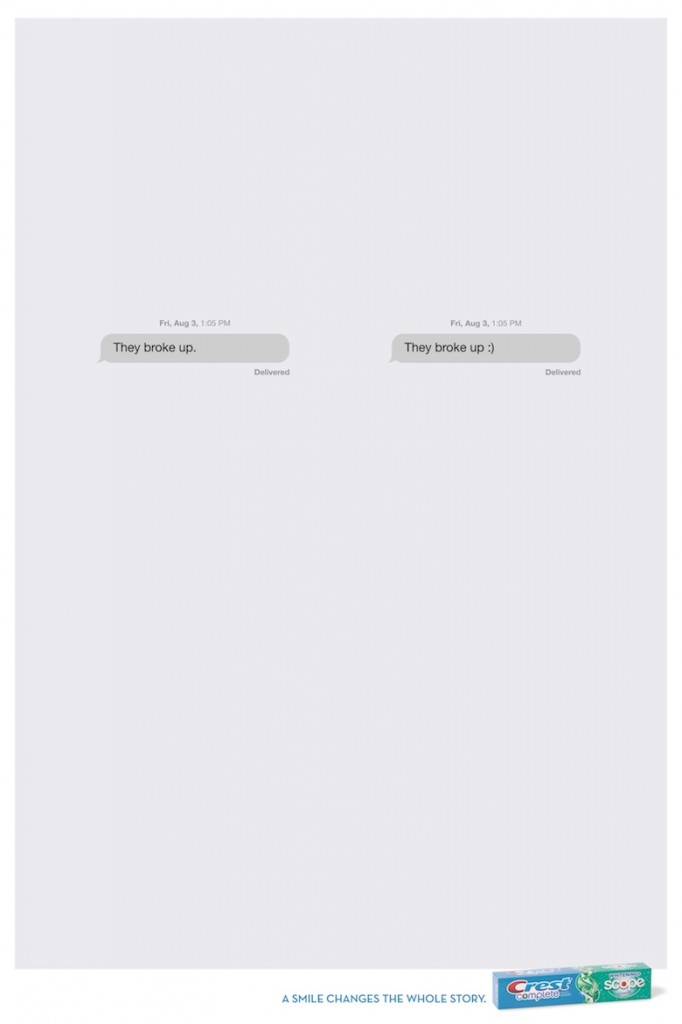In the image, a gray background is divided into ten sections, prominently displaying the date and time: "Friday, August 3rd, 1:05 PM." An oval shape containing the phrase "They broke up" is stamped with the word "Delivered." This is reiterated, showing once again: "Friday, August 3rd, 1:05 PM, they broke up. Delivered."

At the very bottom of the image, a blue checkmark signifies that "A smile changes the whole story." 

Additionally, there is a box featuring various colors: predominantly blue on the left, green on the right, and red text in the middle spelling out the word "Scope." The composition of the text and colors appears to be a nod to branding, reminiscent of Crest Scope toothpaste packaging. The contrasting colors and textual elements provide a thematic representation of change and transformation, suggested by the recurring phrase, "They broke up," and the conclusion that “A smile changes the whole story.”